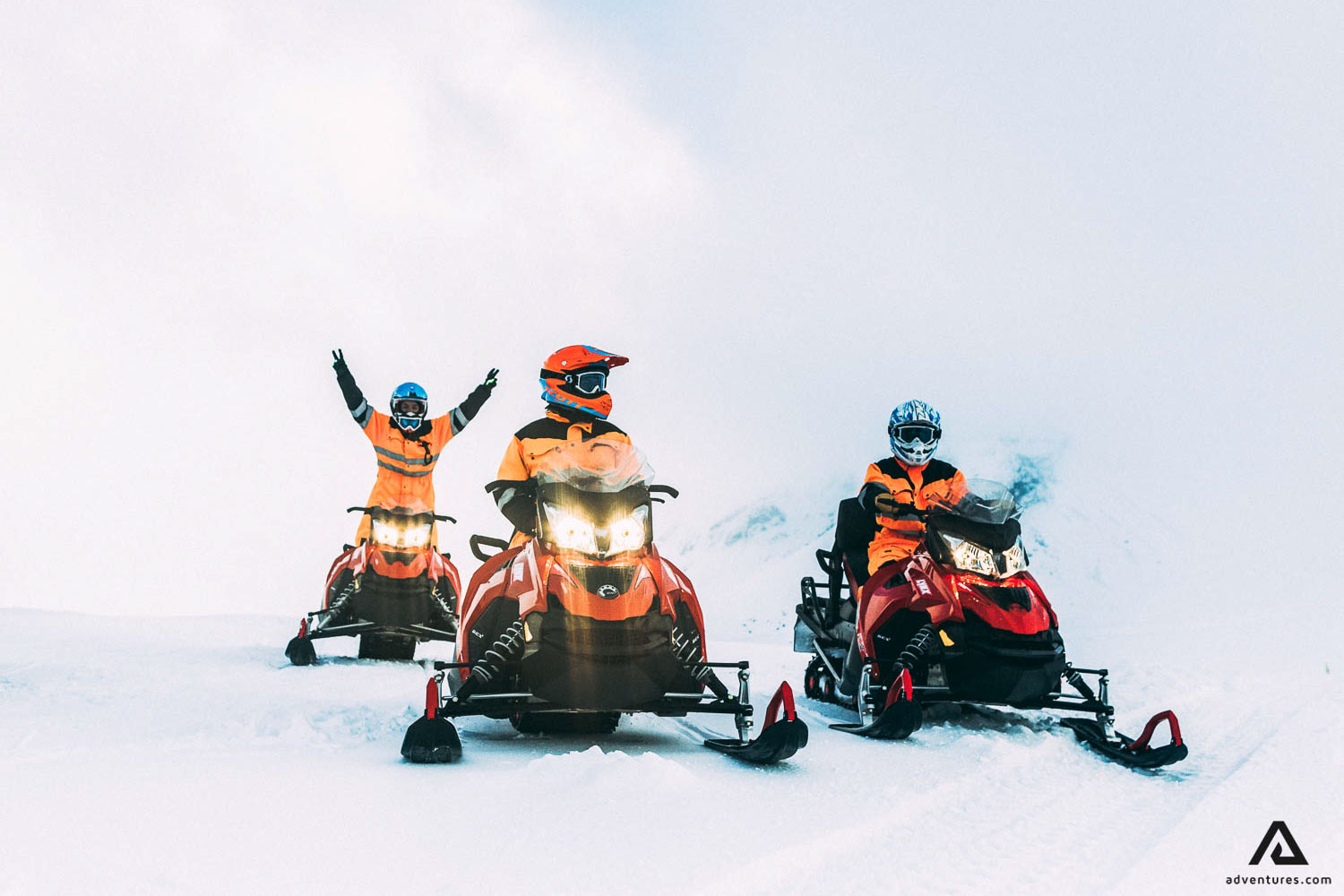The image captures a dynamic winter scene featuring three individuals on snowmobiles set against a predominantly white backdrop of snow and a cloudy sky with slight hints of blue peeking through. The snowmobiles are arranged in a staggered formation, with two in the foreground and one in the background. The snowmobiles have predominantly reddish-orange and red hues with black accents and illuminated yellow headlights. The individuals are uniformly dressed in orange and black winter jackets with helmets and goggles, except for the figure in the background who has his goggles lifted.

In the foreground, one rider in the center, clad in an orange helmet with black goggles, has his hands resting in his lap, while the other rider to the right, wearing a blue and white helmet, grips the handlebars. The most striking figure is the one in the background, standing on his snowmobile, arms raised in a victory pose with peace signs, wearing a light blue helmet and no goggles. The compact snow beneath them and a faint outline of snow-covered mountains add depth to the scene. The bottom right corner of the image features a stylized 'A' logo, accompanied by the text "adventures.com".